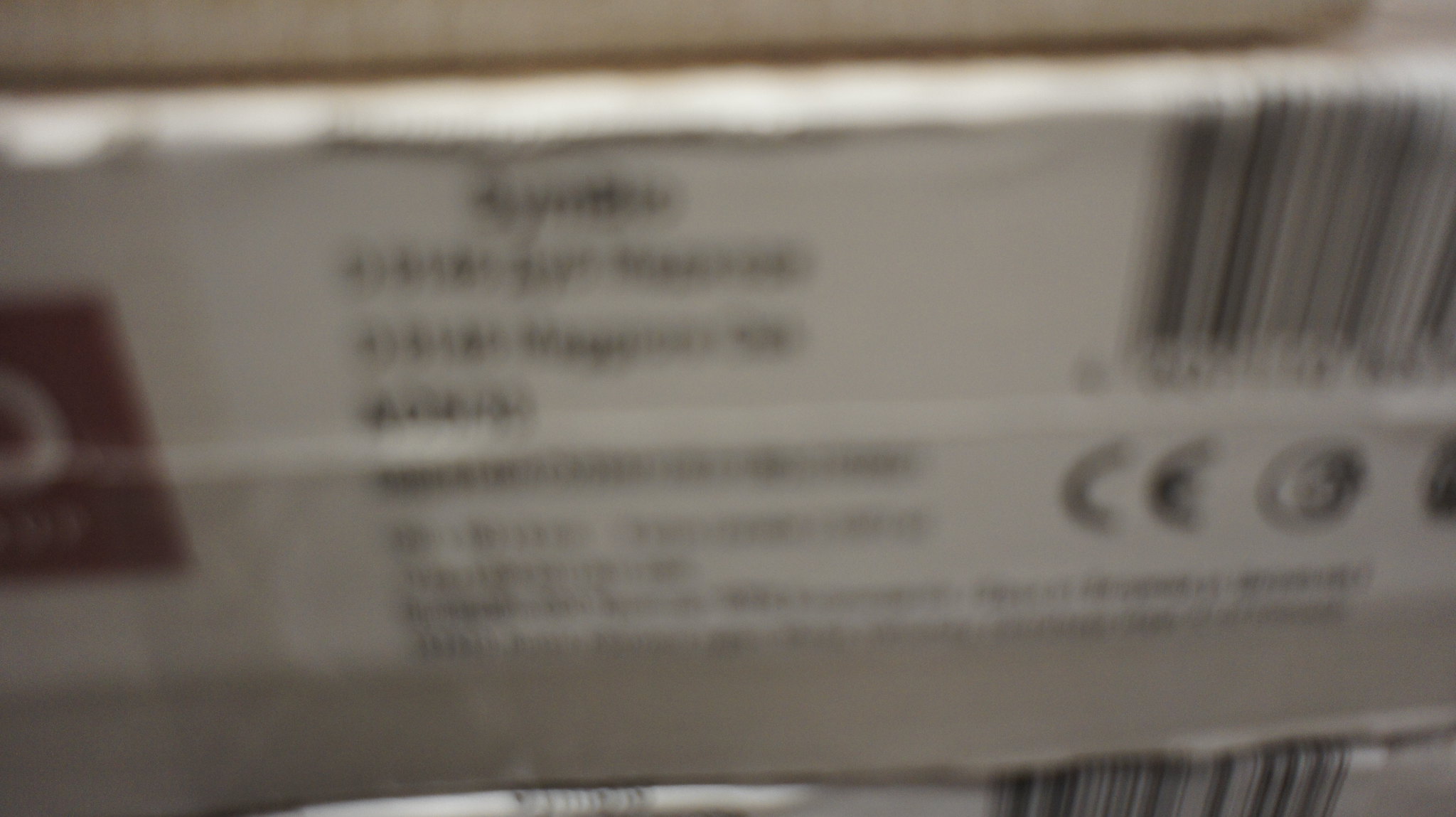A highly blurred, extreme close-up photograph capturing part of an object with a white sticker in the center featuring black text. On the left side of the sticker, there is a partially visible red logo, which appears to be a square shape with a white element inside, though it is cut off and difficult to discern. On the upper right corner of the sticker, a barcode is present, with a series of symbols located directly below it. The background upon which the sticker is placed seems to be a white surface, but due to the blurriness, the exact nature of the object, whether it is a box or an appliance, remains indistinguishable.